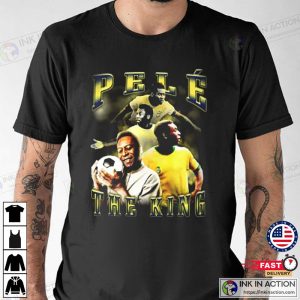The image is a detailed online store listing for a t-shirt featuring the legendary footballer Pele. Central to the image is a heavily tattooed man, though his head is cropped out, showcasing the shirt prominently. The t-shirt is adorned with bold, yellow lettering edged in black shadows that spell out "Pele The King." Below this text are four images of Pele, capturing different moments in his illustrious career, including a recent picture of him holding a soccer ball. 

To the left of the t-shirt, there are icons indicating the available apparel options for this design: a t-shirt, tank top, long sleeve shirt, and a hoodie. The bottom right corner of the image includes several details: an American flag within a small circle, text reading "FAST DELIVERY," and "INK IN ACTION" with a website. This comprehensive listing highlights the versatility and patriotic branding of the apparel.